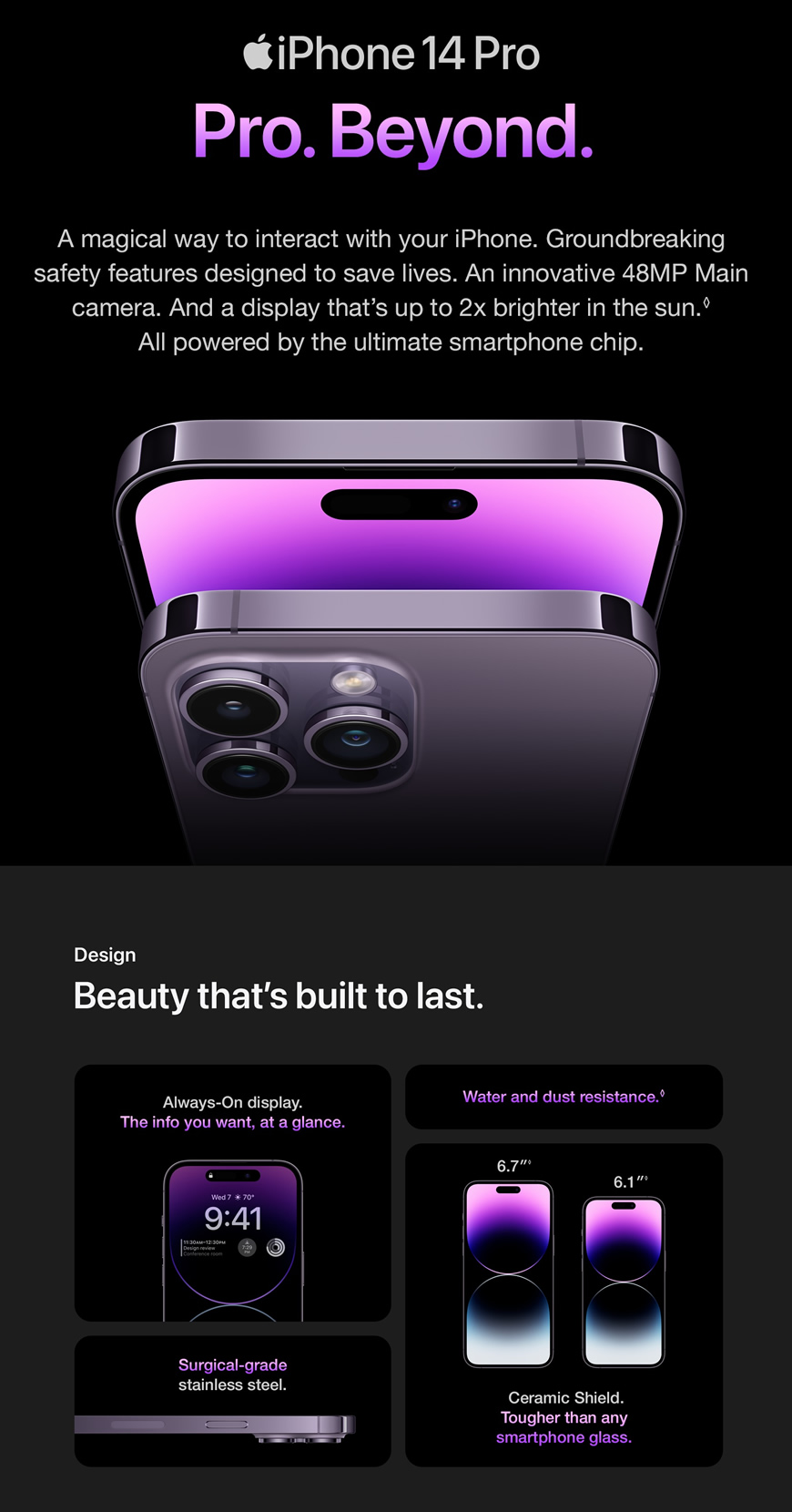The image features a sleek, black background with a prominent white Apple logo at the top, symbolizing the Apple brand. Directly below the logo, the text "iPhone 14 Pro" is displayed, accompanied by the word "Pro" in striking purple text, followed by a period. Further down, the word "Beyond" also appears in purple, completed with a period.

Below this text, a detailed description in white font reads: "A magical way to interact with your iPhone, groundbreaking safety features designed to save lives, an innovative 48 MP main camera, and a display that's up to two times brighter in the sun, all powered by the ultimate smartphone chip."

Centrally, the image showcases a purple iPhone 14 Pro. The phone is prominently featured with its top side and the distinctive triple-camera system visible at the bottom of the frame. Beneath the phone image, another line of white text proclaims: "Design beauty that's built to last."

To the left of the main iPhone image, there is another iPhone displaying the time "9:41." To the right, there are two additional images of the iPhone 14 Pro models, differentiated by screen size: one being 6.7 inches and the other 6.1 inches. These phones feature a gradient color scheme that transitions from light pink at the top, to purple, then to black, and finally to white at the bottom.